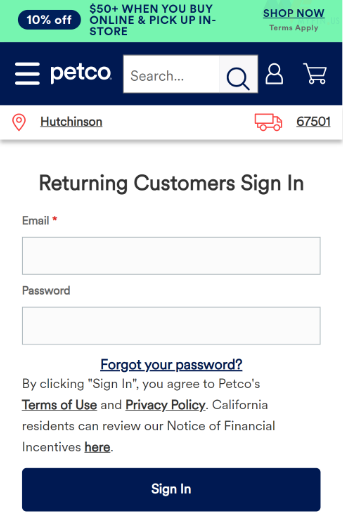The image is a color screenshot displaying the mobile version of the Petco website. At the top of the page, a green banner features a blue oval on the left with "10% off" written in white text. Adjacent to it, blue text reads, "$50 plus when you buy online and pick up in store. Shop now, terms apply." Below this, a dark blue header includes the Petco logo, represented by three white horizontal lines with the word "Petco" in white lettering. The header also contains a search bar labeled "search," a magnifying glass icon, a white silhouette of a person, and a white shopping cart icon.

Next, a white banner with a red location pin indicates the word "Hutchinson" and the zip code "67501," with a red van icon driving to the right. Beneath this, the text "returning customers sign in" is displayed with "email" marked by a red asterisk. There are blank fields provided for entering an email and password. A "Forgot your password?" link is available for users needing assistance. The sign-in section notes, "By clicking sign in, you agree to Petco's terms of use and privacy policy. California residents can review our notice of financial incentives here." Finally, a blue "Sign in" button is positioned at the bottom of this section.